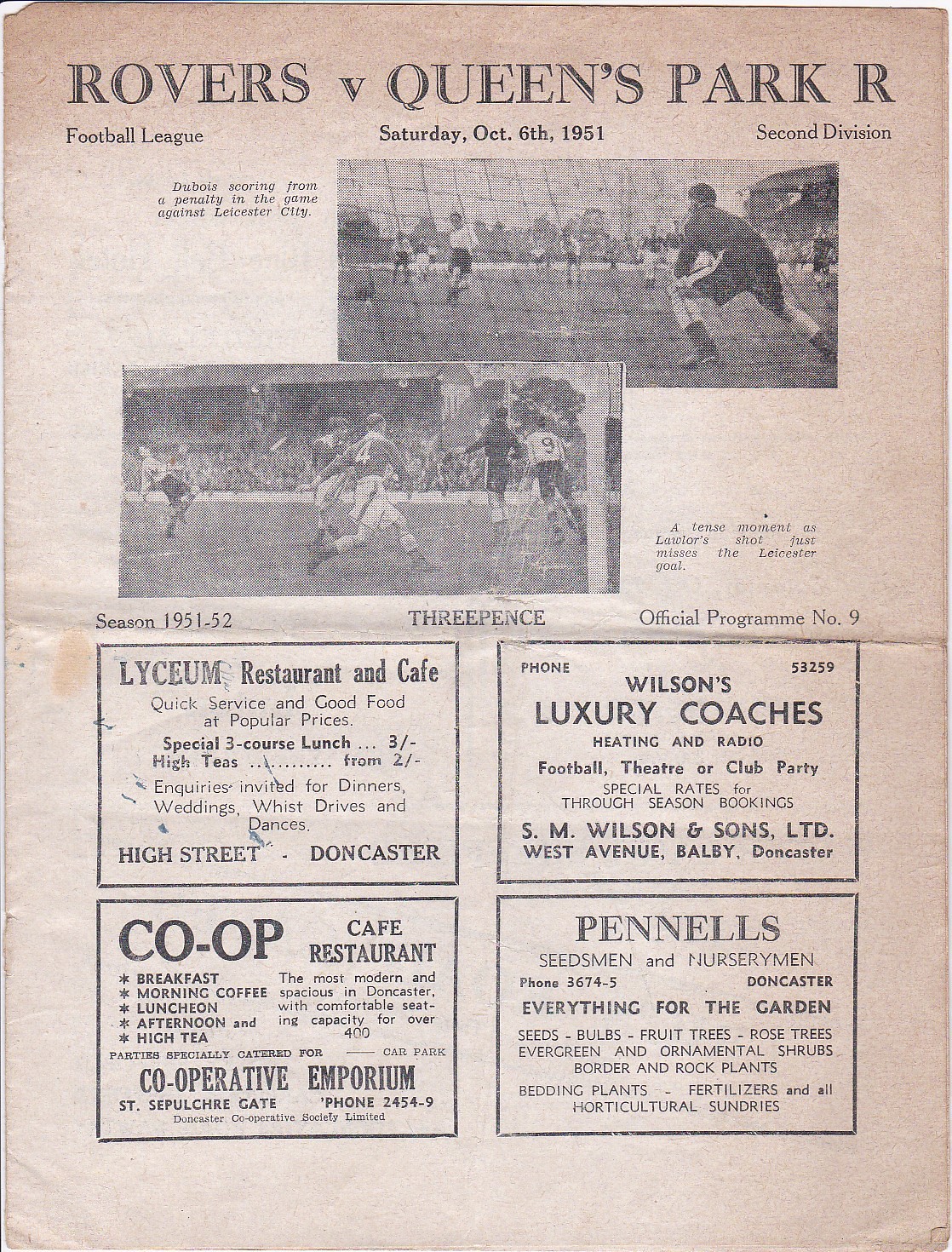This image features a vintage black-and-white printed cover of a soccer program from the UK, dating back to the 1951-52 season. The program is for a second division football league match between Rovers and Queens Park, held on Saturday, October 6, 1951. Bold black lettering at the top reads "ROVERS v. QUEENS PARK R," with "FOOTBALL LEAGUE" in the top left corner, "SATURDAY, OCTOBER 6, 1951" centered, and "SECOND DIVISION" in the top right corner.

The top half of the page showcases two overlapping black-and-white photographs of soccer players in action, including moments like Du Bois scoring from a penalty in a game against Leicester City and a tense scene where Lawler's shot just misses the Leicester goal. Below these images, the text reads "SEASON 1951-52," "THREE PENCE," and "OFFICIAL PROGRAM NUMBER NINE."

The bottom half of the page contains four rectangular advertisements, arranged in a way that forms a larger rectangle. These ads are for sponsors, including Lyceum Restaurant and Cafe, Wilson's Luxury Coaches, Co-op Cafe Restaurant, and Pennell's Seedsmen and Nurserymen, adding a touch of mid-20th-century commercial nostalgia to the program.